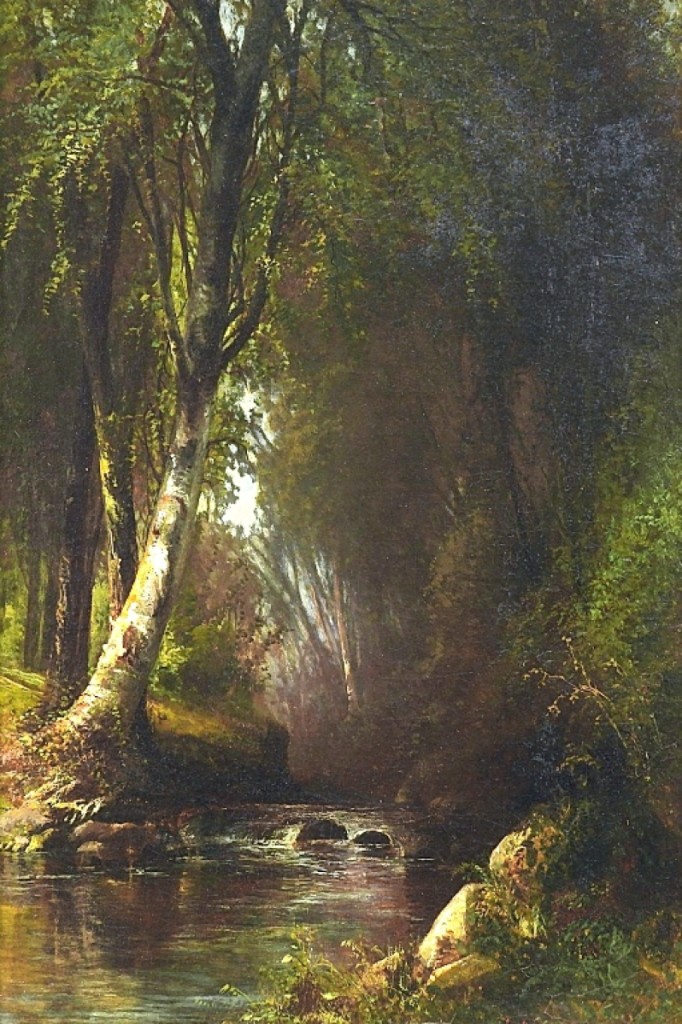This painting, possibly a famous and professionally executed artwork, depicts a serene creek scene set within a dense forest. The vertical orientation of the painting draws the viewer's eye from the body of water at the lower left corner to the dense canopy of trees above. The creek, colored with various purples and greens to suggest reflections of surrounding foliage, winds through the center of the image. A small, frothy waterfall cascades over rocks in the middle of the creek, creating a focal point in the composition. The creek is flanked by tall, dirt shorelines forming small cliffs, adding to the secluded nature of the setting.

Towering trees dominate both sides of the creek, their dark brown and white bark contrasting with the abundant green leaves. Notably, one of the trees on the top right boasts bluish leaves or flowers, adding a touch of unique color to the scene. The artist skillfully captures the play of light filtering through a gap in the branches, creating a striking reflection in the creek. The entire piece, devoid of any text, immerses the viewer in a natural, almost untouched forest landscape, showcasing the artist's meticulous attention to detail and mastery in depicting light and texture.